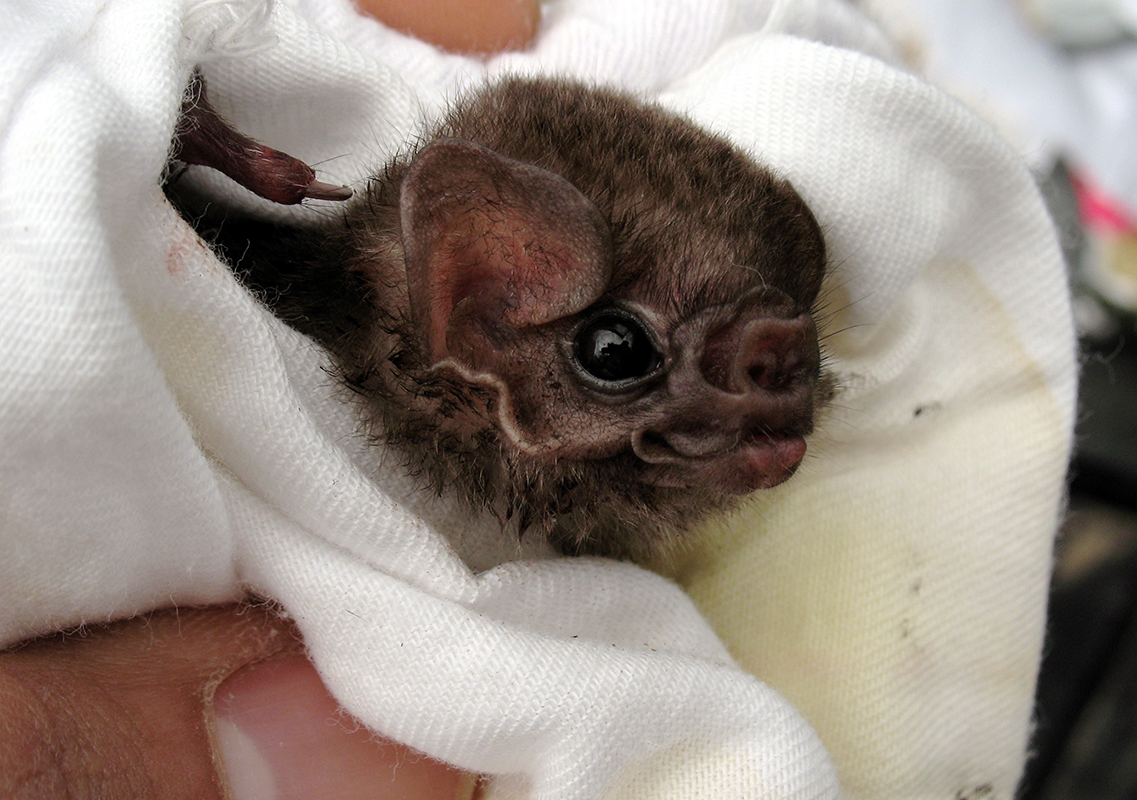In this detailed photograph, a tiny, very young baby bat is being gently cradled in a soft, white cloth held by someone's hand. The bat's head, about the size of the person's thumb tip visible in the bottom left corner, is wrinkled and adorned with patchy fuzz. It has a distinctively wrinkled nose and mouth, as well as a rippled and contoured nose shape. Its large, beady black eyes and oversized ears dominate its small face, giving it an endearing appearance. One of the bat's small claws protrudes from the cloth, pointing to the left. The bat's fur displays a mix of gray and brown hues. The background of the image is blurred, putting the focus squarely on the bat's intricate features and the tender moment it shares with its human caregiver.